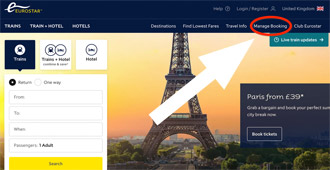The image features a user interface from the Eurostar website. The top portion of the interface is highlighted by a navy blue border with the Eurostar logo in yellow, accompanied by a stylized white "E" with an elongated line extending from its side. Adjacent to the logo, there are options labeled "Train," "Train + Hotel," and "Hotels."

In the top right corner, several buttons are visible: a "Help" button, and buttons labeled "Log In" and "Register." Additionally, there is a "United Kingdom" option with a British flag icon next to it. Below these options, a navigation menu bar is shown including links for "Destinations," "Find Lowest Fares," "Travel Info," "Manage Booking," and "Club Eurostar."

An attention-grabbing red oval is drawn around the "Manage Booking" link, accompanied by a large white arrow pointing towards it. Below the navigation menu, there is a beautiful image of Paris featuring the Eiffel Tower, lush green trees, and distant city buildings in the background. To the left of this image, there is a text box interface for users to enter their travel details, including fields labeled "From," "To," "When," and "Passengers." Below this input section, a prominent yellow button is labeled "Search."